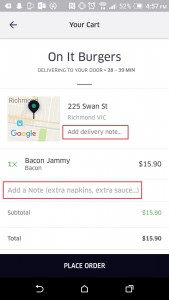![Screenshot of Food Delivery App]

The screenshot showcases a food delivery app interface with various details:

- **Background**: The interface has a clean, white background.
- **Status Bar**: The top status bar indicates a battery level of 52%, the time is 4:57 PM, and there is an alarm clock icon.
- **Header**: Below the status bar, there is a header with a text "Your Cart" and a left-facing arrow.
- **Main Section**:
  - **Food Item**: The screen shows an order for "Tom's Bacon Jimmy Bacon" priced at $15.90.
  - **Delivery Information**: The delivery time is estimated between 28 and 39 minutes.
  - **Map and Location**: A map with a location icon pinpointing "225 Swain Street, Richmond, V.I.C."
  - **Additional Options**:
    - **Add Delivery Route/Note**: There's a prominently outlined red rectangle labeled "Add delivery route/note."
  - **Special Instructions**: An optional note field with the text "(extra napkins, extra sauce)" enclosed within another red rectangle.
  - **Price Breakdown**:
    - **Subtotal**: $15.90
    - **Total**: $15.90
- **Action Button**: At the bottom, there's a prominent blue rectangle containing the white text "Place Order."
- **Icons**: The bottom of the screen displays a reverse arrow, a house icon, and two squares, likely for navigation within the app.

This interface efficiently organizes the user's cart and delivery details for a seamless ordering experience.